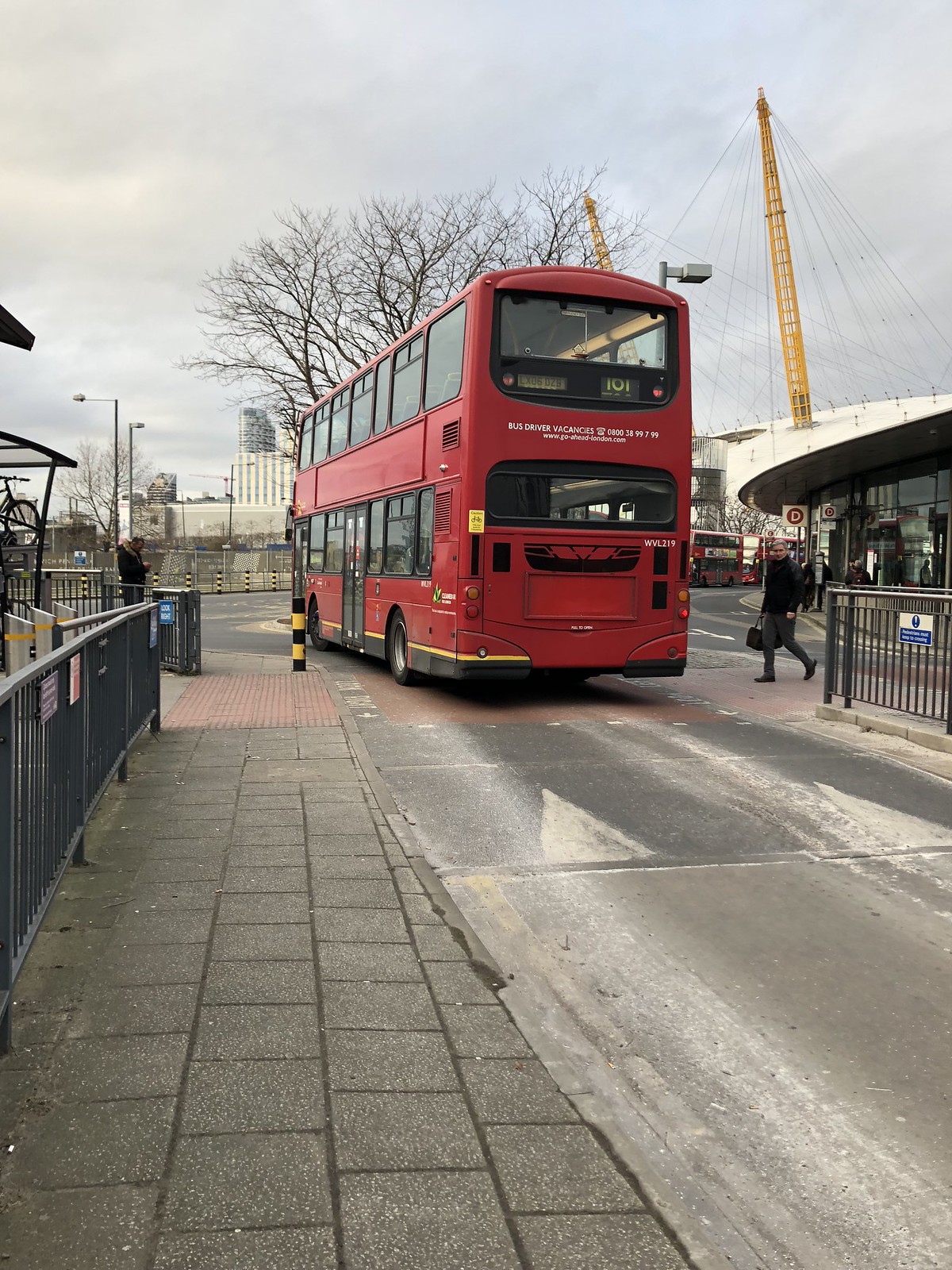This outdoor photograph captures a vibrant street scene featuring a prominent red double-decker bus driving past. The bus, mostly red with white writing advertising driver vacancies, also displays an unreadable yellow sticker on its side. Visible are large windows on both the first and second levels, providing a good view into the bus's interior. On the right side of the image, a man in gray pants and a black jacket, holding a black duffel bag, prepares to cross the street. The street is flanked by gray sidewalks made of square stones and lined with black metal fencing on both sides. In the backdrop, a tall tree devoid of leaves stands against a gray, cloudy sky, alongside distant buildings. Notably, the photograph also hints at a bus depot further down the street, where additional double-decker buses appear to be parked around a curved glass-fronted building with yellow scaffolding-like structures and suspension wires.